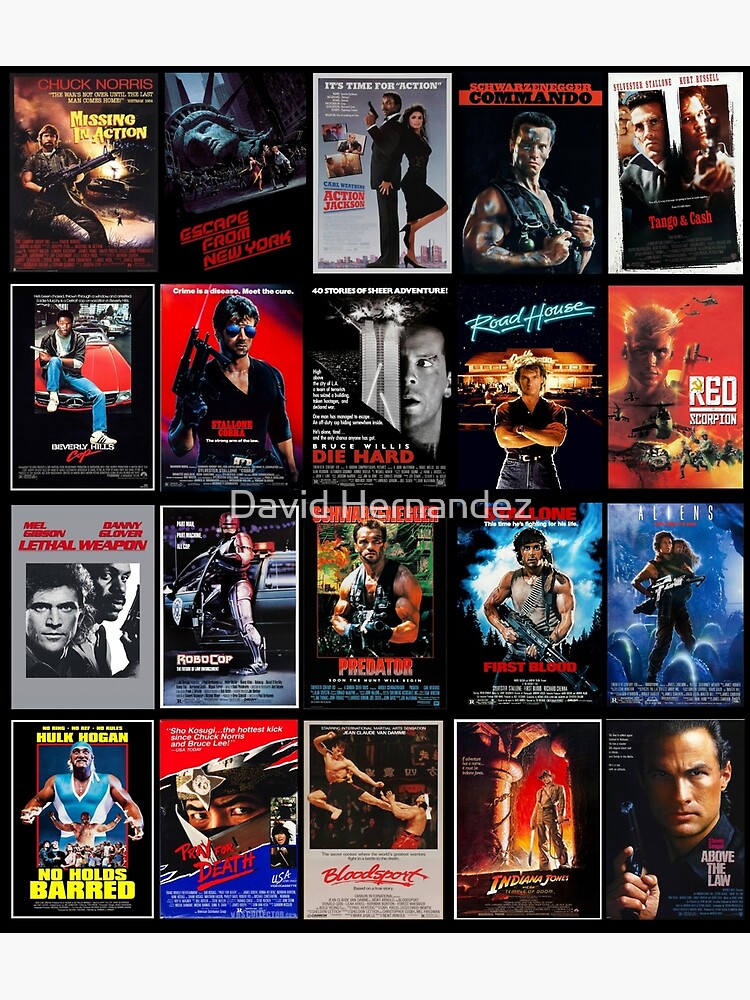The image showcases a vibrant collage of 20 action movie posters arranged in a grid of five columns and four rows. Each individual poster depicts an iconic action film, featuring renowned action stars such as Sylvester Stallone, Arnold Schwarzenegger, Chuck Norris, Bruce Willis, Mel Gibson, Hulk Hogan, and Dolph Lundgren. Highlighted titles include "Commando" with Schwarzenegger in army paint and a sleeveless vest, "First Blood" showcasing Stallone with his M60, "Predator" featuring Schwarzenegger, "Lethal Weapon" starring Mel Gibson, "Bloodsport" with Jean-Claude Van Damme, and "Die Hard" with Bruce Willis. The posters are diverse in color with vibrant red, blue, and yellow hues, each prominently displaying its title and main action hero. This visually striking collection captures the essence of classic action cinema, celebrated by many for their runs in movie theaters and repeated television showings.